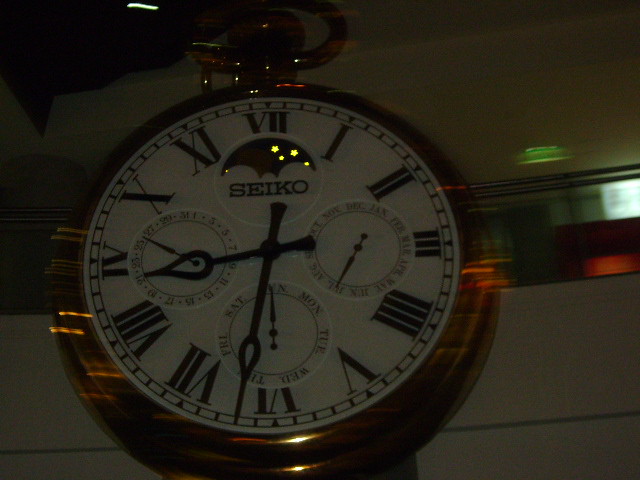This image showcases a sophisticated Seiko watch face encased in a gold frame, exuding an air of timeless elegance. The main dial is adorned with Roman numerals and dominated by a prominent pair of hands at its center. The brand name "Seiko" is elegantly inscribed within a small circle at the top of the dial. The intricate design features four sub-dials, each with its own specific function: the top sub-dial without additional markings, the right sub-dial indicating the month, the bottom sub-dial indicating the day of the week or date, and the left sub-dial displaying numerical counters in odd increments (1, 3, 5, 7, 9, 11, etc.).

Despite the overall blurriness of the photograph, the reflective surfaces of the watch catch the light, creating an interplay of reflections along the sides. The watch is mounted in a dark frame against an indistinct background, which faintly resembles either an interior of a car or perhaps the inside of a refrigerator owing to a silver metallic band traversing the middle of the image.